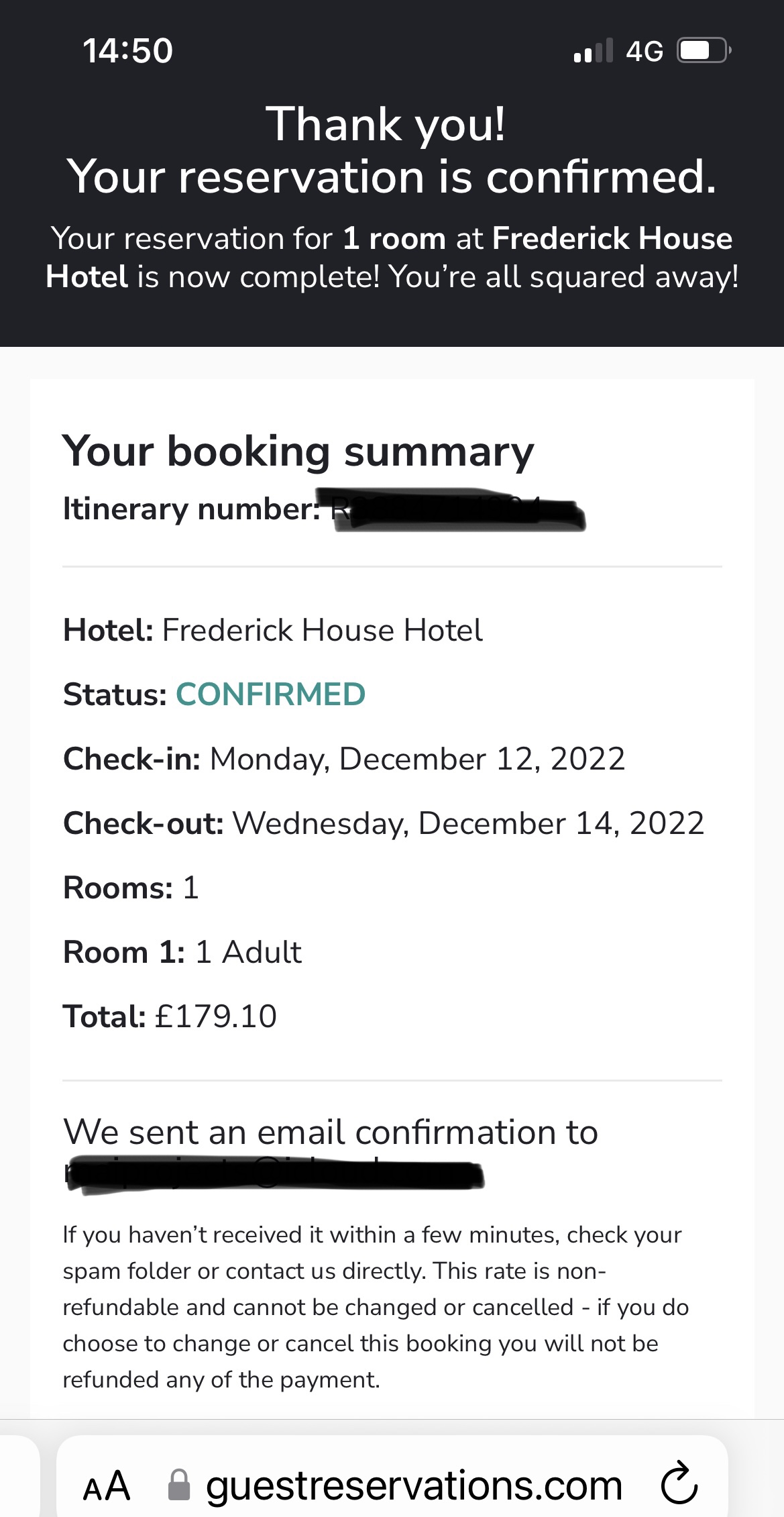Caption:

"This image depicts a smartphone screen displaying a reservation confirmation page for the Frederick House Hotel. The top half of the screen features a black title bar with white text reading, 'Thank you, your reservation is confirmed.' This is followed by a brief message stating, 'The reservation for one room at Frederick House Hotel is now complete. You're all squared away.'

In the body of the page, with a white background and black text, the reservation details are listed methodically. The first line reads, 'Your Booking Summary,' followed by 'Itinerary Number:' with the actual number obscured for privacy. A gray line separates the header from the subsequent information.

The section below presents the specifics of the booking:
- 'Hotel: The Frederick House'
- 'Status: CONFIRMED' (highlighted in teal and all caps)
- 'Check-in' and 'Check-out' dates, formatted as day, month, year.

Further detailed are:
- 'Rooms: 1' indicating the number of rooms booked.
- 'Room 1: 1 Adult' specifying the room type and occupancy.
- 'Total: £179.10' capturing the total cost of the stay.

Below the financial details, a final note indicates that an email confirmation has been sent to the guest's email address, which is blacked out for confidentiality."